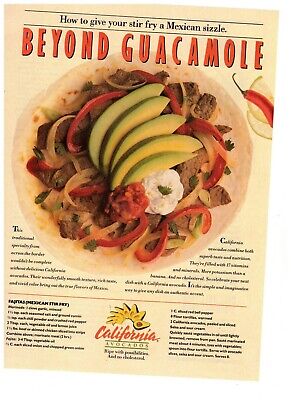The image features a page likely from a magazine or cookbook, showcasing a vibrant and enticing dish under the bold red headline "Beyond Guacamole." Above this title, in black letters, it reads "How to Give Your Stir-Fry a Mexican Sizzle." At the center is a circular photograph of a tortilla generously topped with a colorful array of ingredients: slices of avocado, bell peppers, onions, meat, cheese, salsa, and sour cream, all arranged artfully. On the right side, there is an image of a red jalapeño with a green stem. Below the tortilla, black text is interspersed with small, indistinct writing. Towards the bottom, a red line separates the image from the detailed recipe instructions and the logo "California Avocados," suggesting an endorsement or sponsorship. The vibrant colors and meticulous arrangement of the dish reflect classic Mexican cuisine, designed to entice and inspire culinary creativity.